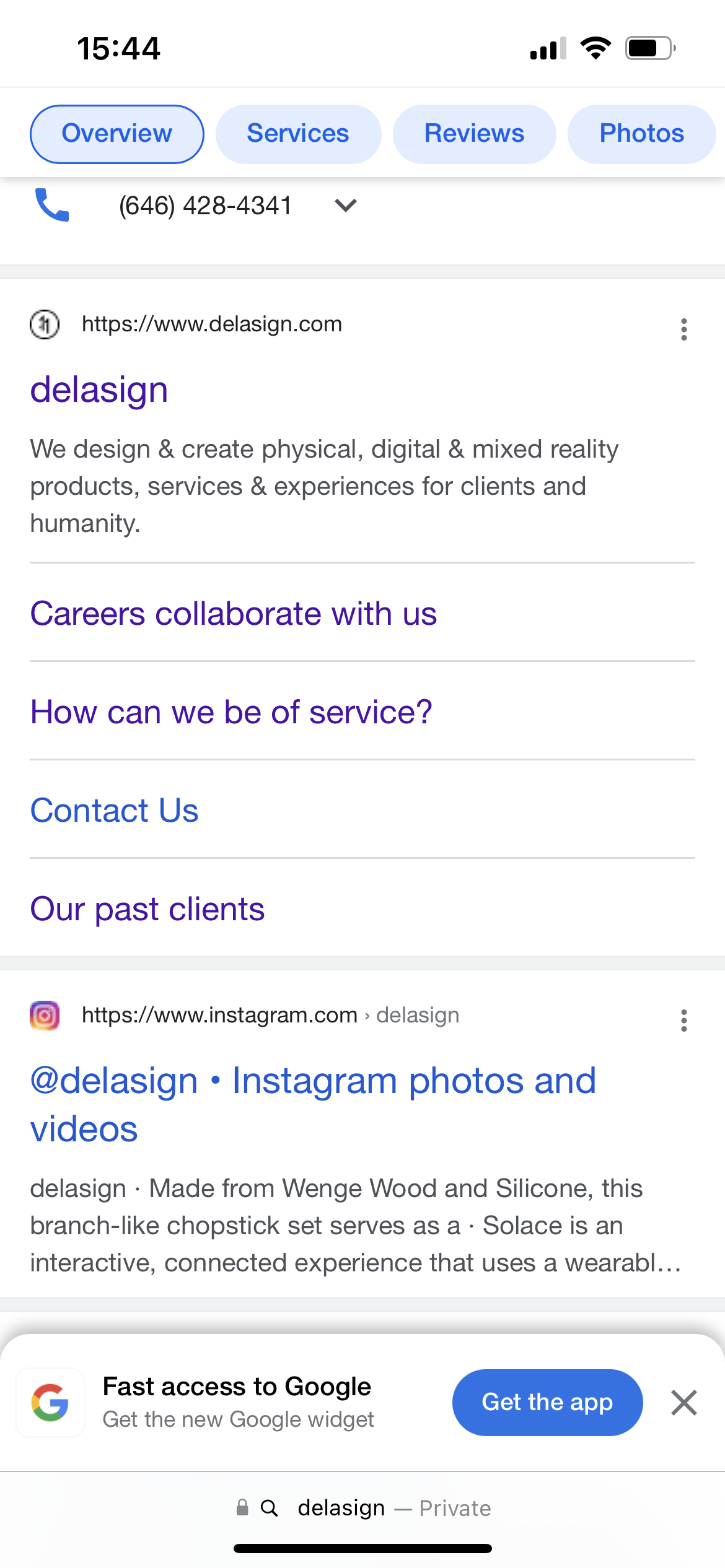The image displays a small portion of a cell phone screen showcasing a website's user interface. On the left corner of the top bar, the number "1544" is prominently displayed, while the right corner features icons indicating cellular signal strength, Wi-Fi connectivity, and battery life.

Below this top bar, there is a light blue navigation strip with options written in blue font: "Overview," "Services," "Reviews," and "Photos." The "Overview" tab is currently active, as indicated by its blue outline.

Further down, there's an icon of a phone followed by the number "646-428-4341" and a drop-down arrow. Beneath this, the URL "delasign.com" is written in blue text. The website seems to be pronounced "Delasign," and it focuses on designing and creating physical, digital, and mixed reality products, services, and experiences for clients and the general public.

The section below offers several options, separated by thin gray lines: "Career Collaborators," "Careers," "Collaborate with Us," "How Can We Be of Service," and "Contact Us." A thicker gray line separates these sections from the subsequent content.

Following this, there is a clickable link, "instagram.com/delasign," leading to Delasign's Instagram page which features photos and videos. Underneath, there is a descriptive caption stating, "Made from Wenge wood and silicone, this branch-like chopstick set serves as a solstice," hinting at one of the products showcased on their Instagram account.